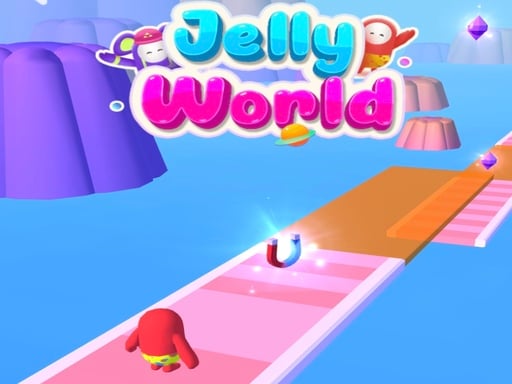The image is a vibrant, animated scene from a video game advertisement called "Jelly World." The central logo, in a playful, childlike font, floats at the top with 'Jelly' in blue and 'World' in pink. Surrounding the logo are round, animated creatures featuring white circular faces and simple black eyes, one with large rounded ears. The scene is colorful and bright, featuring a spectrum of hues like purple, blue, orange, pink, red, green, and yellow. Two notable landscape features are a towering purple structure on the left and an array of floating pathways and bridges hovering above a serene blue ocean. These paths are pink and orange, adding to the whimsical scenery. On one of these pathways, a red, squishy creature wearing yellow shorts heads towards a glimmering, U-shaped magnet that alternates between red and blue with light sparks. The background is filled with fantastical elements, including mountainous islands in shades of purple and pink, jello molds, and twinkling purple diamonds, making the scene appear cheerful and inviting.